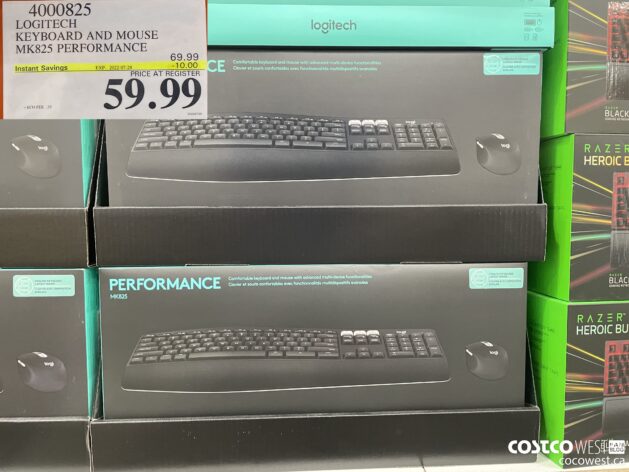This photograph showcases a display of various keyboards for sale in a retail setting, likely a Costco given the pricing and branding details. At the forefront are several gray boxes featuring Logitech keyboards, prominently labeled with the model designation "Performance MK825." The front of each box displays an image of the keyboard itself, in addition to a computer mouse included in the set. The prices and discounts are clearly visible in the upper left-hand corner; originally priced at $69.99, the set now retails for $59.99 thanks to an instant savings offer of $10. The item number for this Logitech keyboard and mouse combo is 4000825.

Adjacent to the Logitech display are more stacks of boxes, partially visible on the right. These boxes are labeled "Razer Heroic" and have bright green sides, suggesting another brand of computer peripherals, possibly gaming keyboards, are also being offered. At the bottom of the photograph, there is a web address, CostcoWest.CocoaWest.ca, indicating that this display might be from a Costco in California or associated with Costco’s West Coast operations.

The overall layout of the display is orderly, with two fully visible Logitech boxes and partially visible ones on either side, providing a clear, albeit segmented, view of the available inventory.